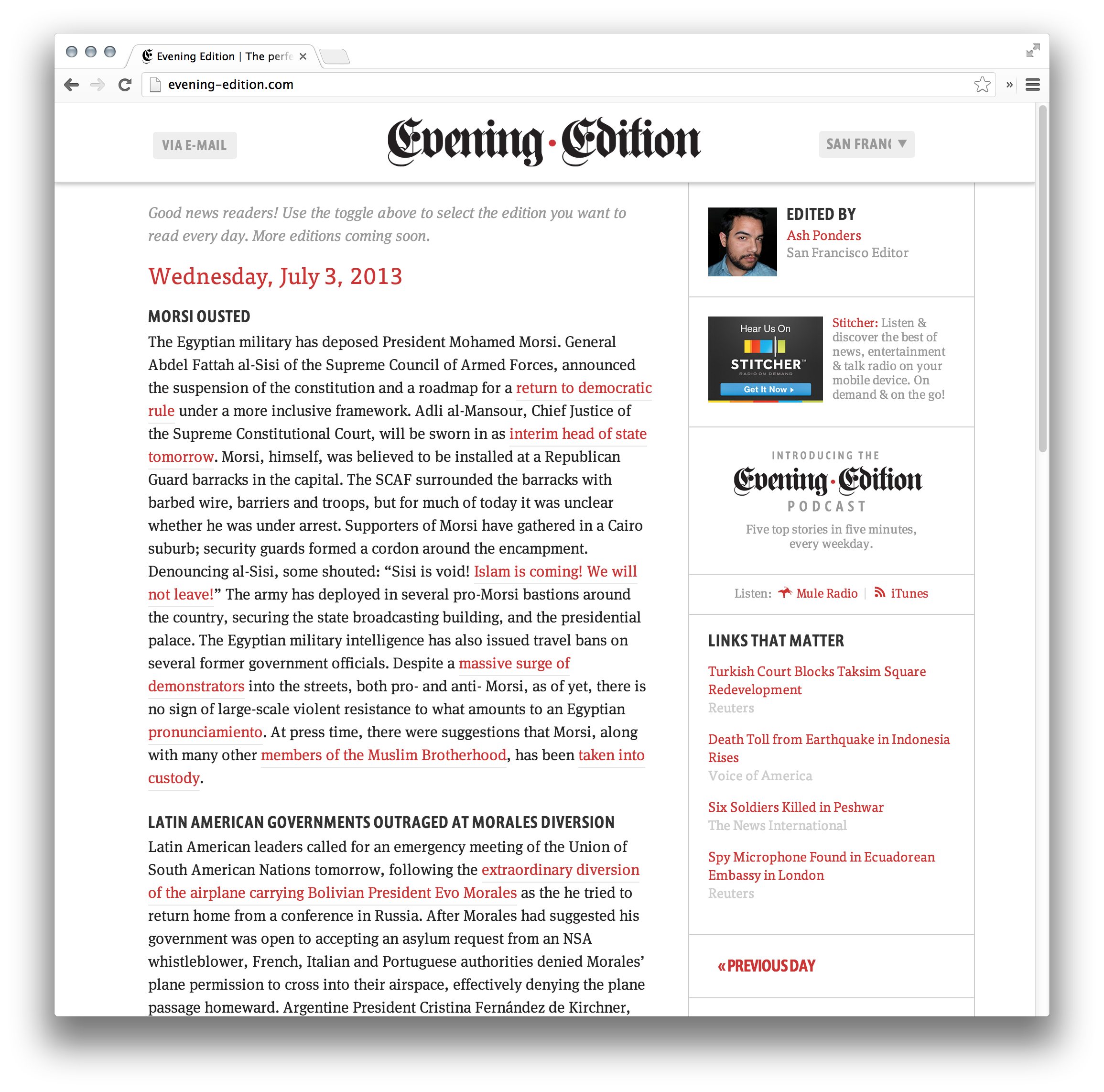This screenshot captures the homepage of the website EveningEdition.com as it appeared on Wednesday, July 3rd, 2013. At the top center, the words "Evening Edition" are prominently displayed in bold. To the left, there is an email link, and to the right, a dropdown menu labeled "San Fran." Below this heading, the text reads: "Good News Readers. Use the toggle above to select the edition you want. Read every day. More editions coming soon."

The main content includes two prominently featured articles. The first article is titled "Morsi Ousted," and the second article is titled "Latin American Governments Outraged at Morales Diversion." The text within these articles is written in black and red fonts.

To the right of the main articles, there is a photograph of the editor, Ash Punders, who is based in San Francisco. Below Ash Punders' photo is an advertisement for Stitcher that encourages users to "Hear us on Stitcher. Get it now."

Under the Stitcher advertisement, additional information introduces the Evening Edition podcast, which delivers "5 top stories in 5 minutes every weekday." Options for listening via Mule Radio or iTunes are provided.

Below this, another section labeled "Links that matter" features the following headlines:
- "Turkish court blocks Taksim Square redevelopment"
- "Death toll from earthquake in Indonesia rises"
- "6 soldiers killed in Pesroi"
- "Spy microphone found in Ecuadorian Embassy in London"

The page also includes a navigation option to view articles from the previous day.